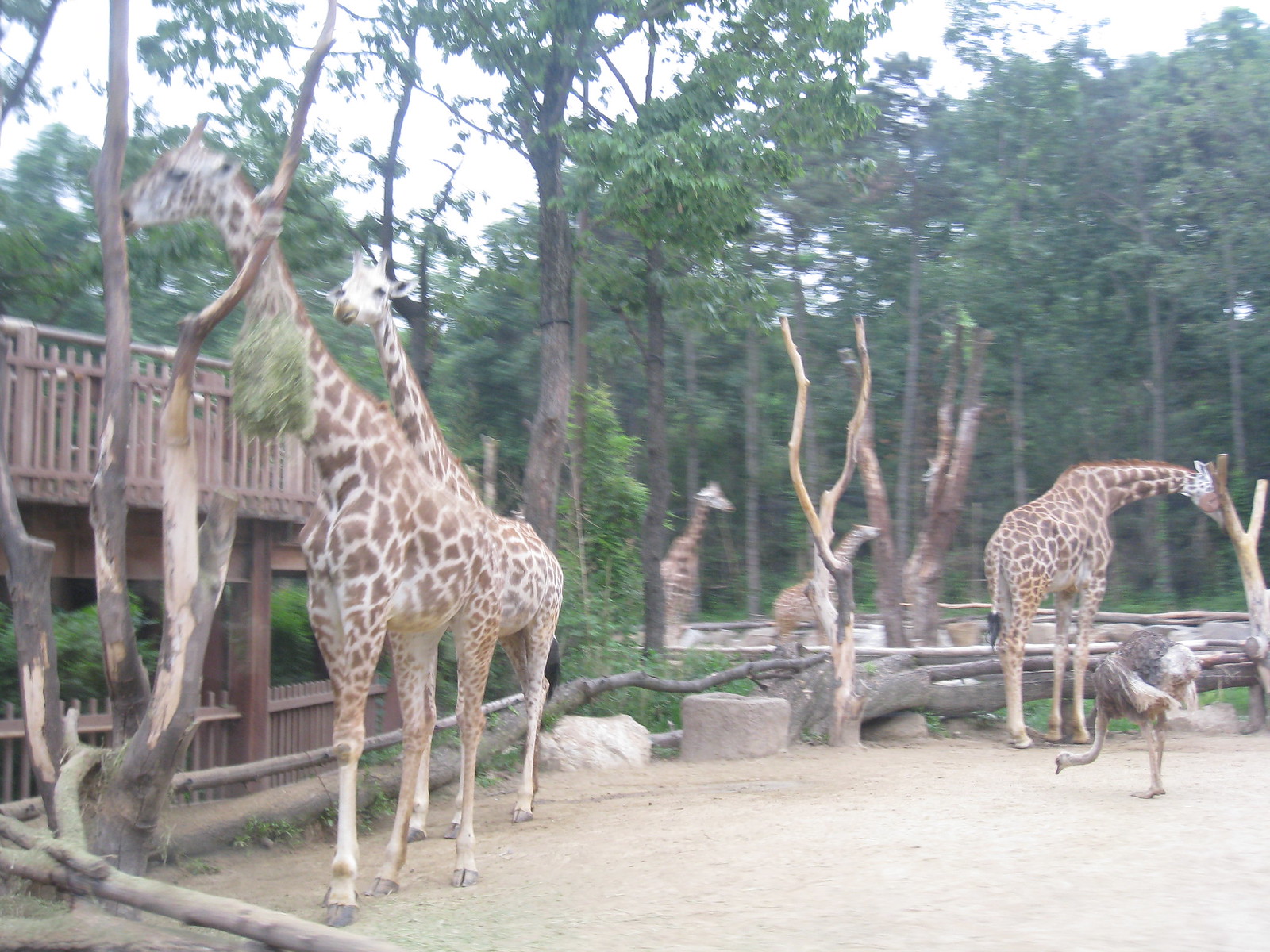This photograph, taken at a zoo on an overcast day, features several giraffes and an ostrich amidst a blurry and low-quality setting. In the foreground, the closest giraffes appear in motion and blurry. The giraffes in the very back of the image are also indistinct, blending into a background filled with trees and wooden pillars. To the left of the photograph, a fenced-in wooden platform supports an enrichment hay holder hanging from a tree. One giraffe, positioned to the left, has its head against the tree, while another giraffe in the middle background looks out aimlessly. On the right side, a giraffe stands behind an ostrich that is pecking at the brown ground, its gray feathers tipped with white. High wooden pillars, large rocks, and green-leaved trees are scattered throughout the enclosure.